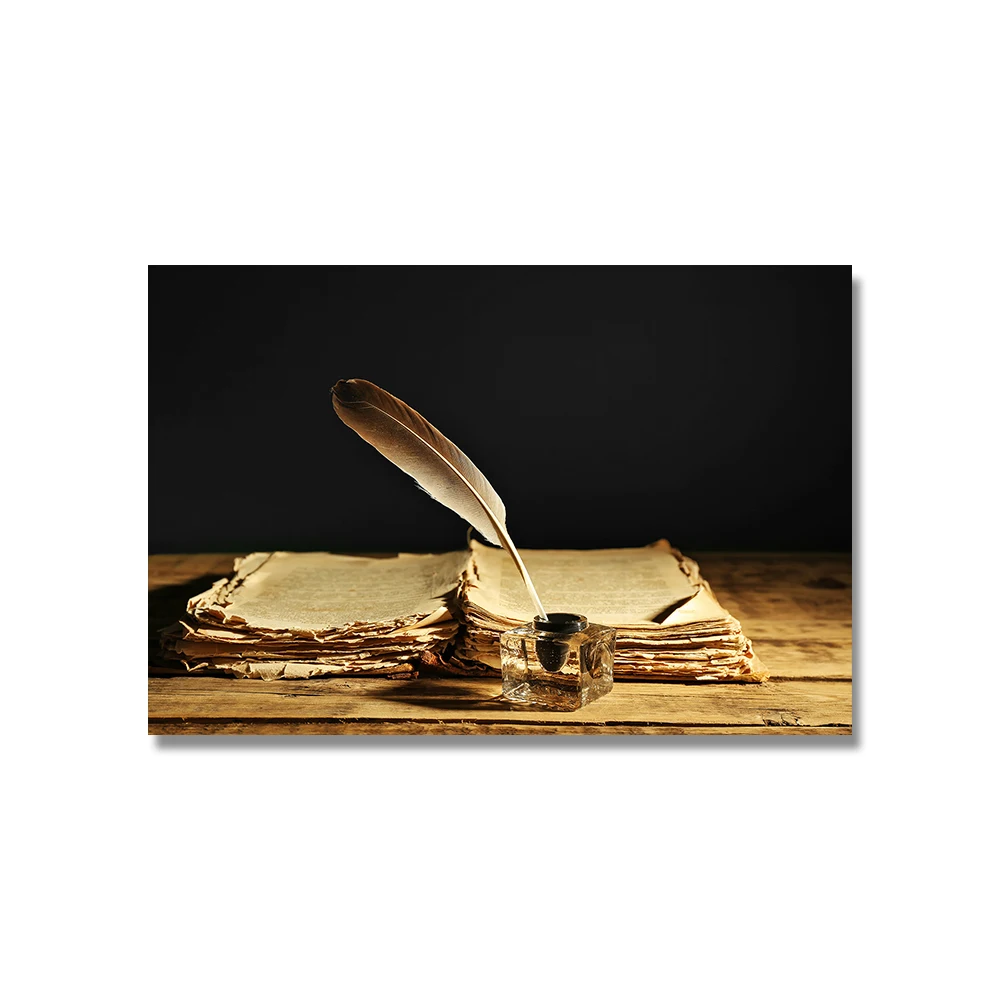In the image, a square full-color photograph taken indoors with artificial lighting, you see a striking scene centered on a collection of aged, tattered papers, possibly attached by fine thread. These ancient, worn pages are stacked on what appears to be an old wooden table, its grain and wear visible despite a backdrop of pure blackness that engulfs the rest of the scene. Dominating the center of this tableau is a clear glass inkwell, almost resembling an ice cube, with a black core of ink. Inside the inkwell sits a feather quill pen, poised and ready as if awaiting to inscribe onto the fragile leaves of paper beside it. The colors in the image are primarily shades of brown, black, grey, and white, reflecting the venerable nature of the objects captured. Despite the presence of writing on the paper, the angle of the photograph obscures any attempt to discern its content, leaving an air of mystery and historical curiosity. There are no people or additional text visible, keeping the focus solely on the timeless objects themselves.